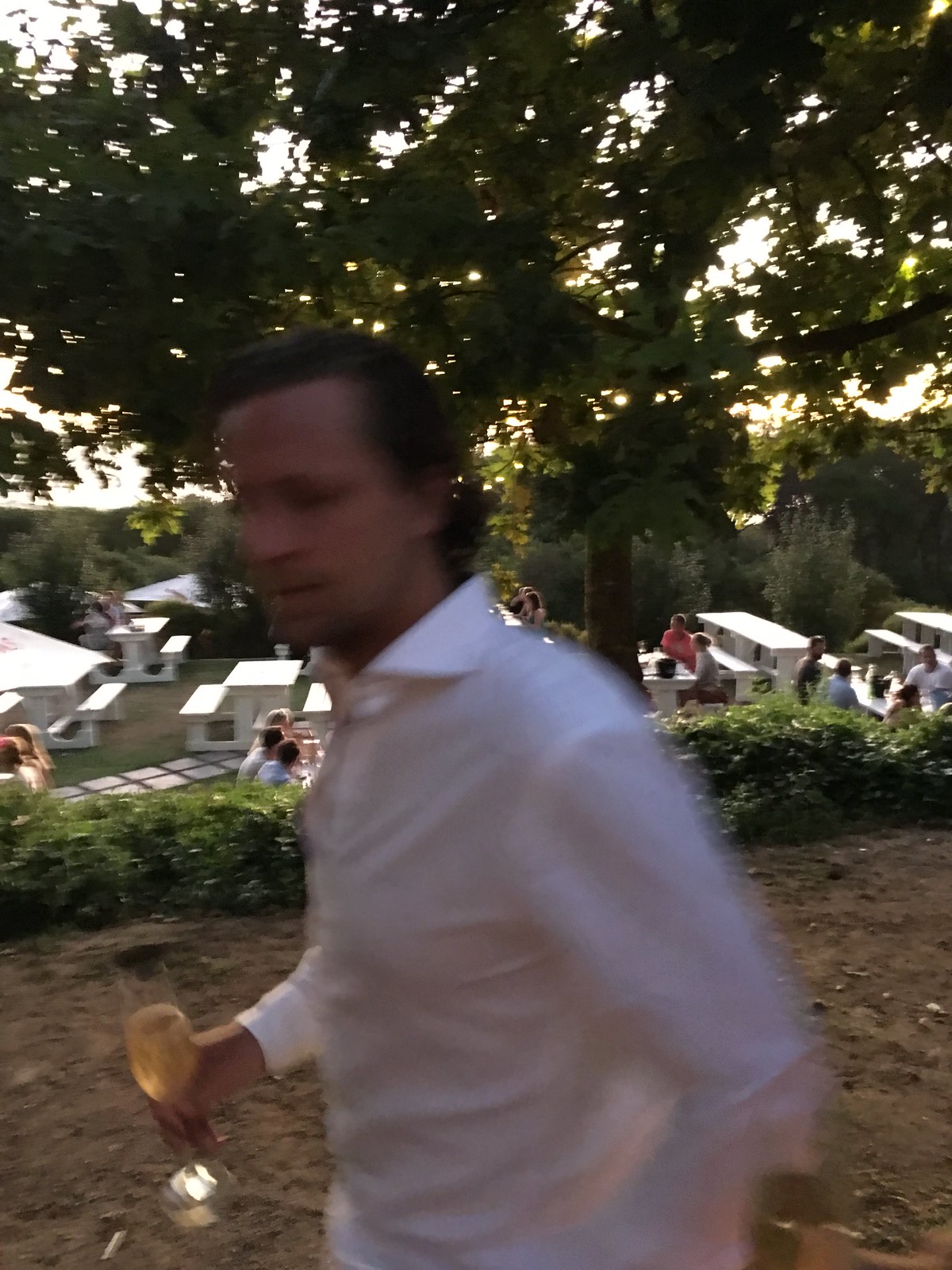This close-up side view captures a man with short, slicked-back brown hair, clad in a long white dress shirt with angular, triangle-like collars. He is holding a champagne glass in his left hand, brimming with bubbly champagne. The effervescence of the drink is visible as tiny bubbles on the surface. The man is slightly out of focus, appearing to be in motion. In the background, people can be seen walking around, with several white picnic tables set up, suggesting a relaxed outdoor gathering. The foreground features a mix of grass and bushes, while a large tree dominates the top of the photo, its branches bathed in the golden glow of a setting sun, casting a serene, warm light over the entire scene.